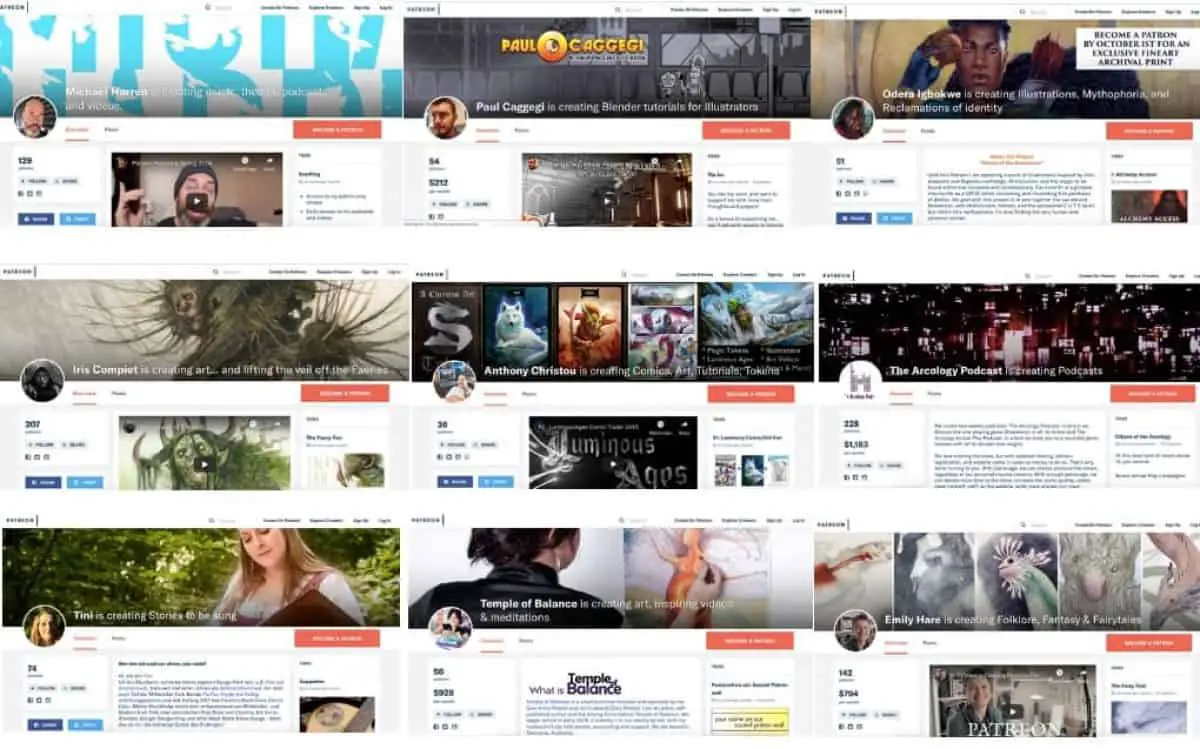The webpage displays a 3x3 grid of individual profiles, each occupying its own section on the page. Each profile encompasses a uniform layout that starts with a banner image spanning the top half. Beneath this banner, positioned on the far left, is a profile picture of an individual, followed by their name to the right of the picture. Each profile includes several components: metric and tracking data on the left, a central video clip, and additional content or details on the right. While the exact purpose of the page remains unclear, it appears to be a compilation of different personal or thematic sites, each meticulously organized for easy navigation and information retrieval.